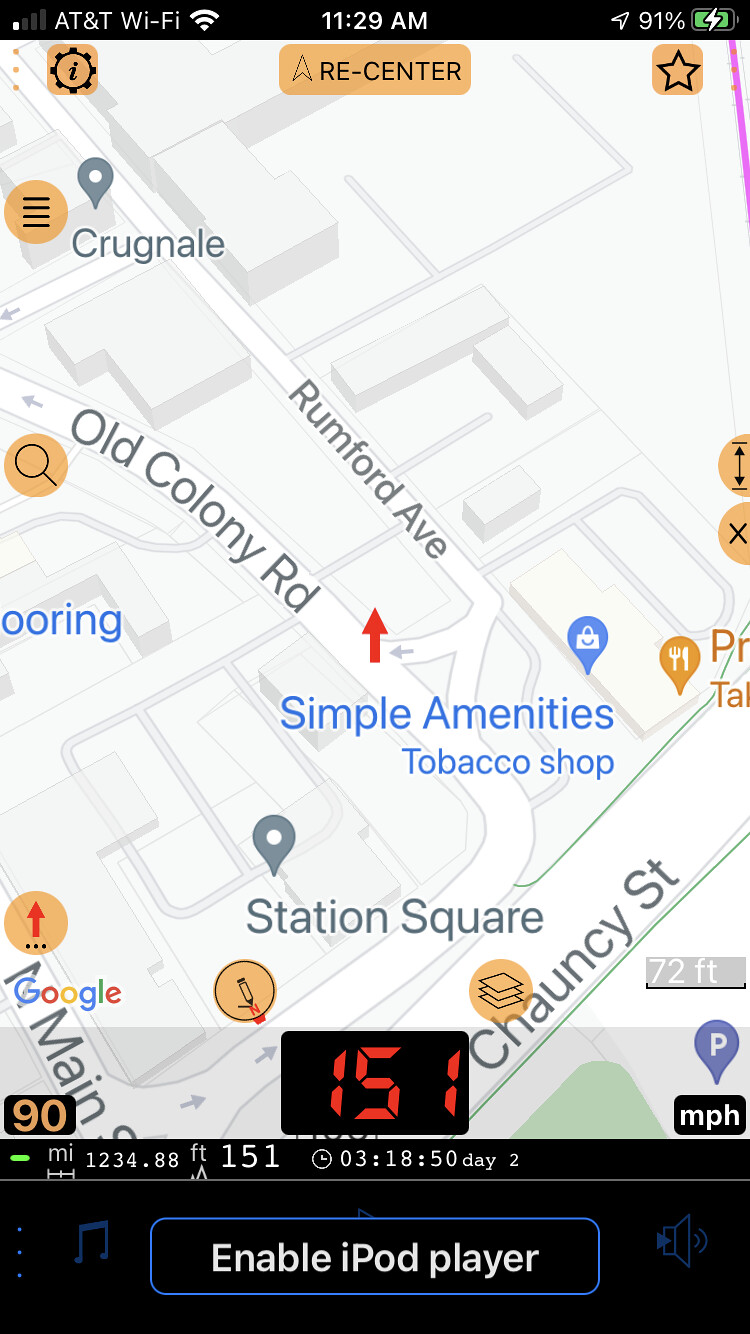This rectangular screenshot captures a map application displayed on a smartphone. The dimensions show that the left and right sides are longer than the top and bottom sides. At the very top, a black banner spans from left to right across the entirety of the image. 

Starting on the left of the banner, there are four ascending signal bars with the first bar white and the subsequent three gray. Following this, white text reads "AT&T Wi-Fi" next to an icon featuring a downward-pointing triangle composed of three curved lines. Centrally placed on the black banner, the time is displayed in white text as "11:29 AM." Towards the right, white text reads "91%" and is accompanied by an icon of an outlined battery that is green and displays a white lightning bolt on it, indicating the battery is charging.

The main portion of the screenshot is a map characterized by gray and dark gray hues, adorned with various labels in blue, gray, and black. The map labels include: "Krungnail," "Runford Ave," "Old County Rd," "Simple Amenities," "Tobacco Shop," "Station Square," and "Chauncey Street." Another label is partially visible, only displaying the letters "-O-O-R-I-N-G," suggesting that the full word is cut off from view.

This caption provides detailed insights into the content and elements displayed within the image.